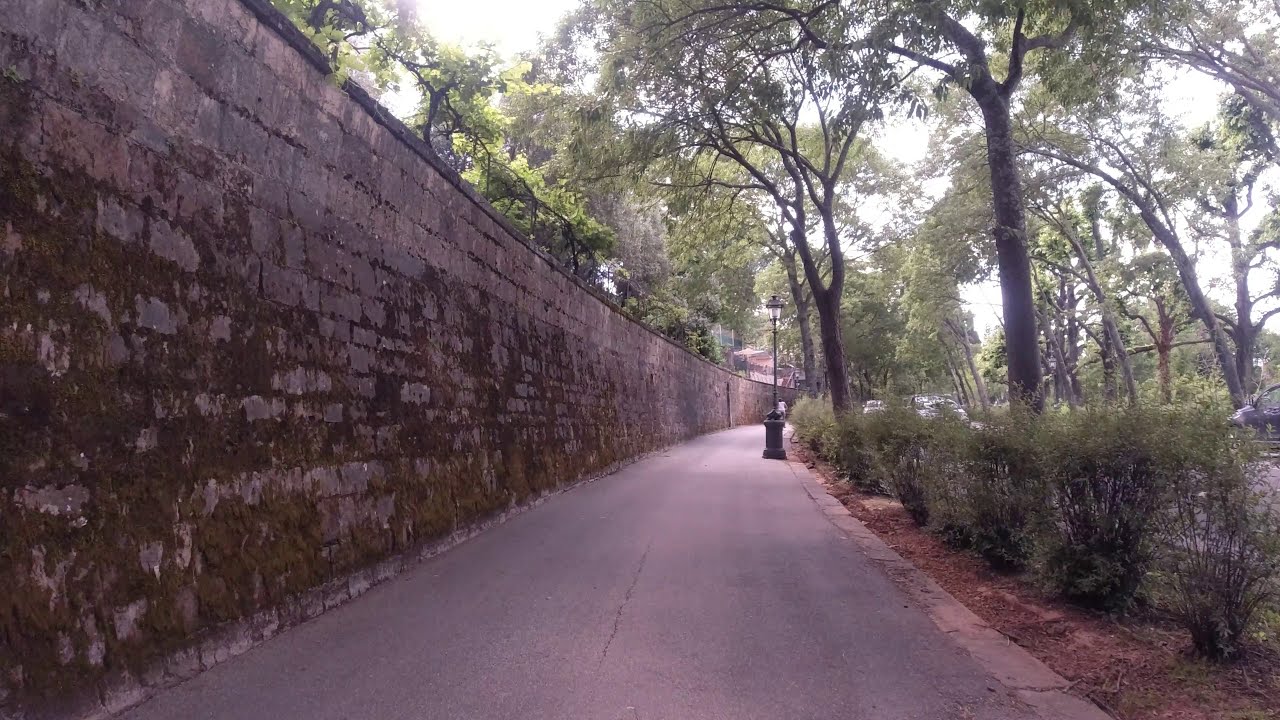The image depicts a serene pathway with dark gray pavement extending from the bottom center and receding into the distance. On the left side, a towering stone wall, approximately 20 to 30 feet high and covered in moss along its bottom two-thirds, runs parallel to the path. The stonework of the wall consists of large gray rectangular stones, and tall green trees rise above it, forming part of the leafy canopy that covers the entire area. To the right of the pathway, the scene is lined with a park-like setting filled with bushes, shrubs, and hedges, along with towering trees that feature brown trunks and leafy green canopies. A dark lamppost with a clear lantern top stands about halfway down the path. Beyond the shrubs on the right, the presence of a roadway becomes evident with a few visible vehicles. Overall, the image showcases a peaceful, naturalistic scene under a canopy of trees with light filtering through a hazy sky.